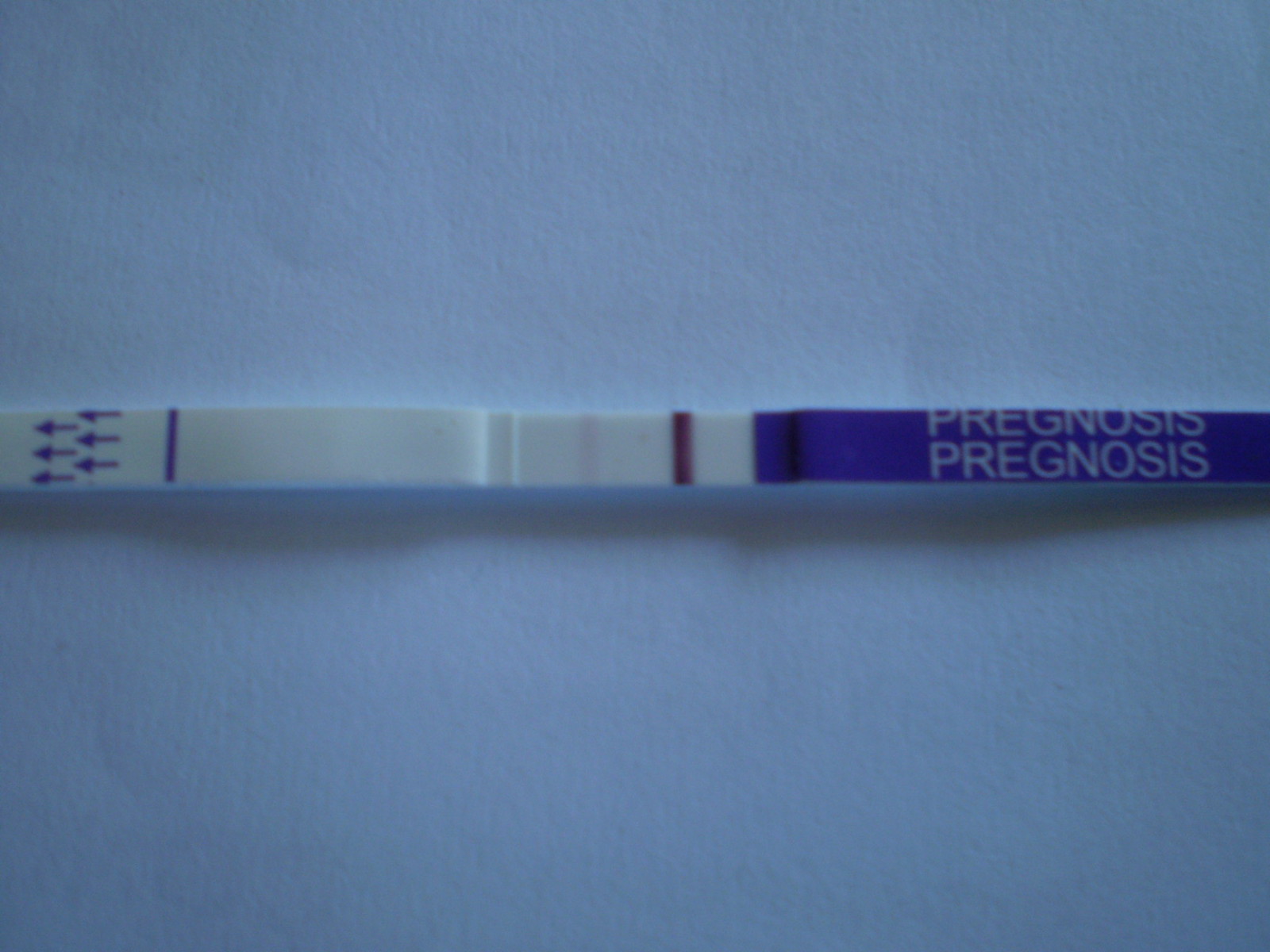The photograph captures a single test strip resting on a slightly wrinkled white sheet of paper, which adds a subtle texture to the image. The paper has a bluish-grayish tint, and a gentle shadow cast by the test strip emphasizes its presence. The overall image quality is somewhat pixelated, making the details appear grainy.

The test strip itself is long and narrow. One end of the strip is a striking royal blue, adorned with white text that reads "PREGNOSIS." Moving towards the middle of the strip, there is a white indent displaying a prominent, purple-blue line. Beside this, a faint second line can be discerned. At the opposite end of the test strip, there is a small section of white followed by a tiny navy line, accompanied by several small navy arrows pointing adjacent to it.